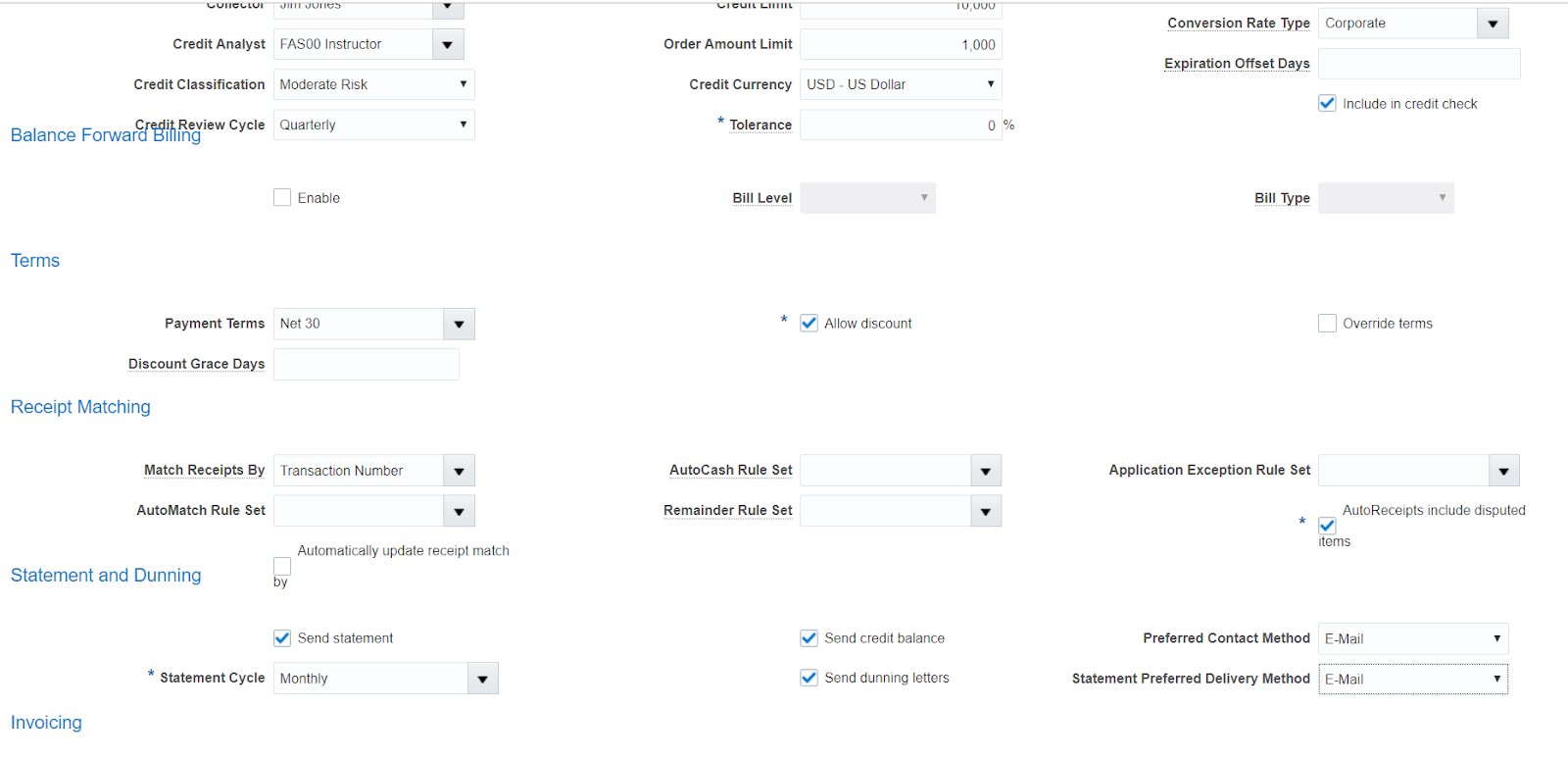The image shows a large page with cut-off top and bottom sections, structured into three columns designed for adding information. 

### Left Column:
- **Title:** Credit Analyst
- **Role:** FASOO Instructor (drop-down menu)
- **Credit Classification:** Moderate Risk
- **Credit Review Cycle:** Quarterly
- **Billing:** Balance Forward Billing
- **Options:**
  - Enable (checkbox, unchecked)
  - Terms, Payment Terms (drop-down menu): Net 30
  - Discount Grace Days (empty box)
- **Receipt Matching:**
  - Matching Receipts by Transaction Number (drop-down menu)
  - Auto Match Rule Set (drop-down menu, empty)
  - Automatically Update Receipt Match (checkbox, unchecked)
- **Statements:**
  - Send Statement (checked)
  - Statement Cycle: Monthly
  
### Middle Column:
- **Order Amount Limit:** 1,000 (currency not specified)
- **Credit Currency:** U.S. Dollars
- **Tolerance:** 0%
- **Bill Level:** (drop-down menu, empty)
- **Options:**
  - Allow Discount (checked)
  - Send Credit Balance (checked)
  - Send During Letters (checked)

### Visual Design:
- The site features a color scheme of blue, black, white, and gray.

The detailed layout offers various fields and options, mostly accessible through drop-down menus and checkboxes, providing a comprehensive interface for managing credit and invoicing details.